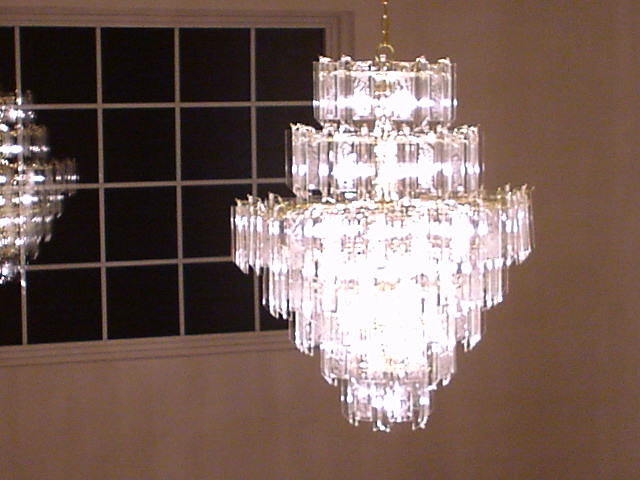In this image, a striking chandelier is the focal point, featuring seven elegant tiers that alternate in size. The top two tiers are smaller, followed by one large central tier, and then four smaller tiers beneath it. The chandelier is adorned with sparkling crystals that catch the light, giving it a radiant glow. Suspended mid-air, it dangles from a gold chain link attached to the ceiling. Behind the chandelier, there is a white-framed window with 20 panes, reflecting the chandelier’s shimmering lights and suggesting it is dark outside. This window contrasts against a tan wall, adding warmth to the setting. The image appears to have been taken inside a room, possibly in a multi-level house, as inferred from its grand placement and reflective surroundings. Despite a slight blur in the photo, the chandelier's intricate details and the ambient night setting are clearly discernible.